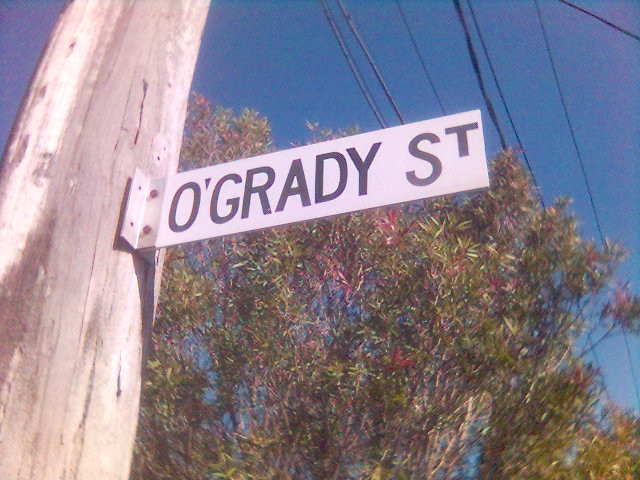On a bright, sunny day with a completely blue sky, power lines and telephone lines stretch above. To the left, a worn and weathered telephone pole stands, its surface transitioning from a lighter brown to an almost gray color. A tall tree reaches up towards the power lines, adding a touch of nature to the scene. Attached to the pole with rusted nails is a street sign in bold black lettering. The sign reads "O'GRADY ST" in all capitals, but notably, the 'T' in 'ST' is positioned higher next to the 'S,' creating an unusual and striking detail.